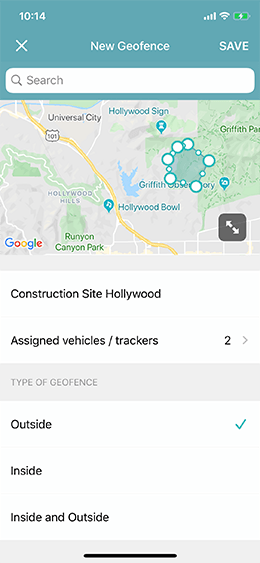A screen capture from a smartphone is shown, with the top left corner displaying the time as 10:14, and the top right corner indicating four bars of cell signal, active Wi-Fi, and a battery at 100% charge. The background features a teal-colored banner at the top. Below this banner is an "X" on the left, the text "New Geofence" centrally located, and the word "Save" on the right. 

Directly below, there is a white search bar that concludes the teal-colored banner. Below the search bar, a detailed map of the area near the Hollywood Bowl is visible, including landmarks such as Universal City, Highway 101, and Runyon Canyon Park. A large green circle with numerous white dots indicates the geofence area, which seems to encompass part of Griffith Park.

Further down, the screen displays the label "Construction Site Hollywood," with the next line reading "Assigned vehicle/trackers to" accompanied by a red arrow. The subsequent line, "Type of geofence," presents three options: "Outside" with a checked green checkmark, "Inside," and "Inside and outside," both of which are unchecked, indicating the geofence being set up is for the outside area only.